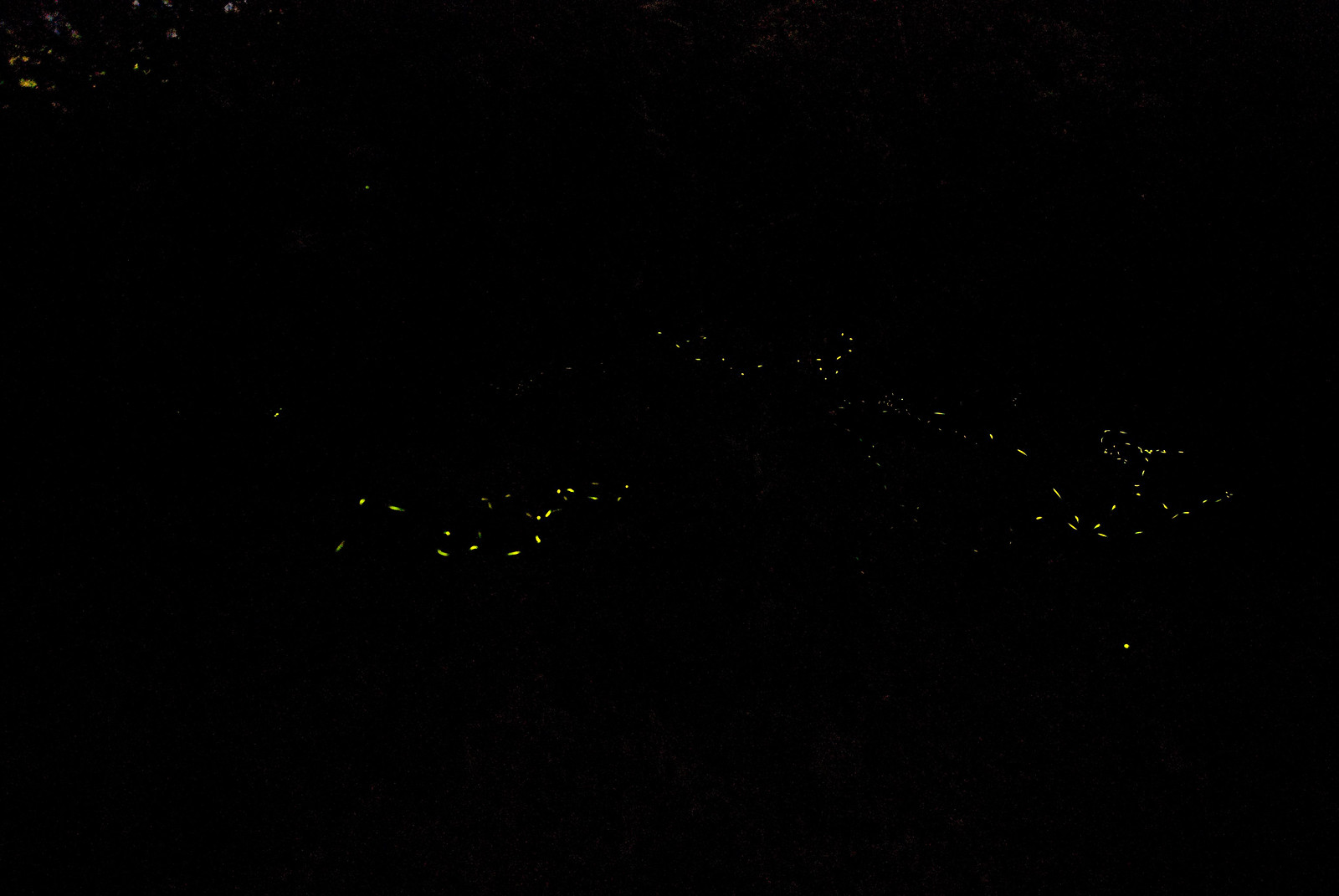The image is a top-down view of a city at night, captured in an almost entirely pitch-black frame scattered with approximately 60 to 70 random yellow dots, representing the lights of buildings. These dots, varying in size and shape, create an irregular and swirling pattern concentrated mostly in the center and a few in the upper left corner of the image. The rest of the photograph, especially the bottom and majority of the top, remains solid black, devoid of any illumination. The randomness of the lights suggests a cityscape seen from a high vantage point, but it's ambiguous enough that it could also be abstract or a digital rendering. There is no text or additional colors present in the image, enhancing the stark contrast between the luminous yellow specks and the deep black background.